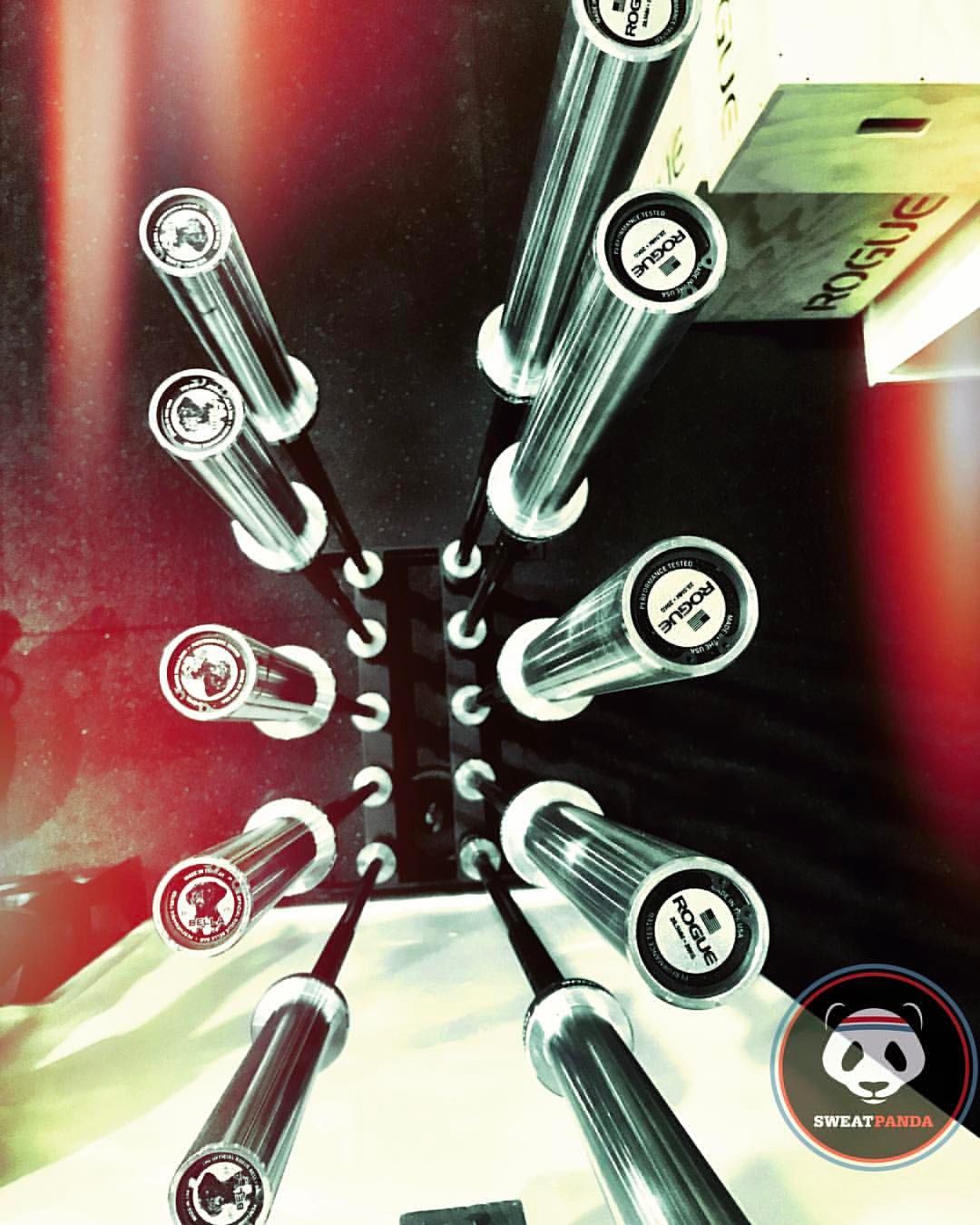This is a computer-generated, color image presented in portrait format, depicting a top-down view of workout equipment arranged on a dark, black and red-tinted background. At the top right corner, there is a wooden box bearing the "Rogue" logo in red text. Central to the image are ten barbell poles, five aligned on each side, housed in a black metal rack. These poles, silver in color, have thicker cylindrical tops that resemble handlebars, each marked with the "Rogue" logo in black. In the bottom right corner, a prominent "Sweat Panda" logo featuring a panda bear with a red, white, and blue headband is visible within a circular background. The visual details and branding elements suggest this could be promotional material for a fitness brand or gym equipment.